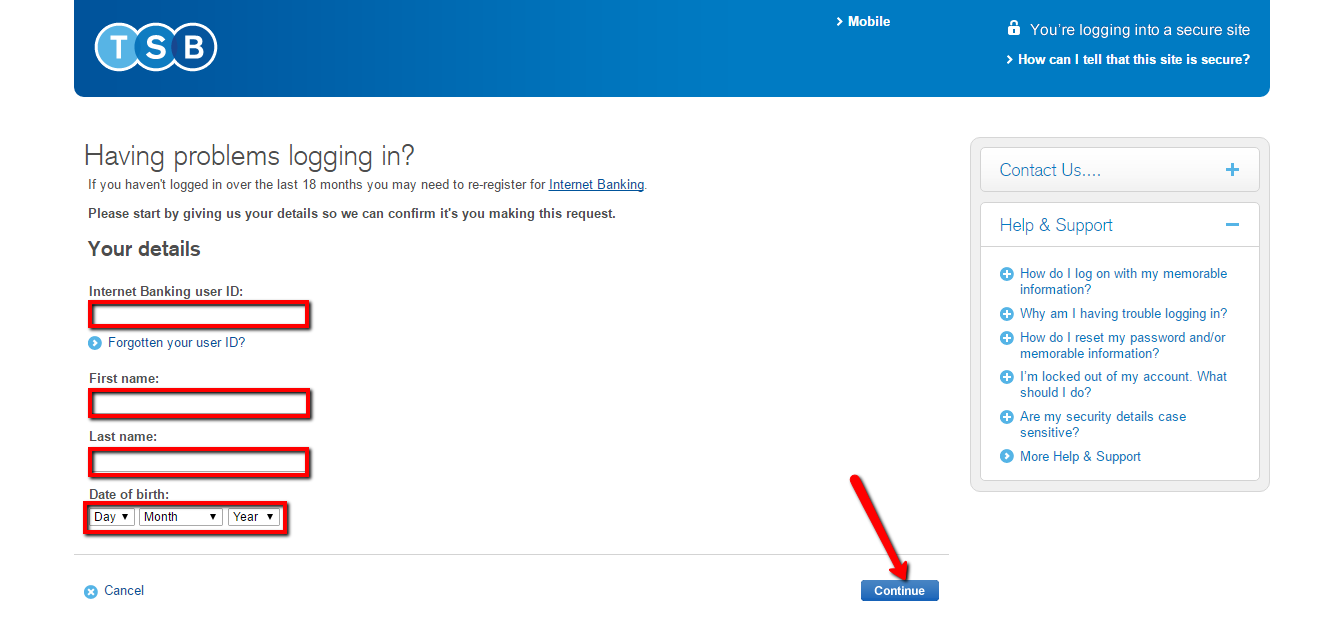This image features a white background with various user interface elements, most prominently dominated by a large blue header at the top. Within this header, the initials "TSB" are displayed in white letters inside individual blue circles. Adjacent to this is a right-pointing arrow with the word "Mobile," followed by a lock icon and a statement indicating that the user is logging into a secure site. Additionally, there's a right-arrow labeled "How can I tell this site is secure?" beneath the lock icon.

Below the header, on the white background, text in blue and underlined informs the user about potential login issues: "Having problems logging in? If you haven't logged in in the last 18 months, you may need to pre-register for internet banking." Following this notice, an instruction is provided: "Please start by giving us your details so we can confirm it's you making this request."

The form below this instruction includes several fields for user data:
- "Your Details" heading
- "Internet Banking User ID" field framed in red with a small blue circle and white arrow beside it bearing the phrase "Forgotten your user ID?"
- "First Name" and "Last Name" fields, both outlined in red
- "Date of Birth" field divided into day, month, and year, all outlined in red

At the bottom of the form, there's a white button featuring a blue circle with an "X" and text that reads "Cancel."

On the right-hand side of the image, a blue box contains contact options:
- "Contact Us" with a plus sign
- "Help and Support" with a minus sign
- Additional clickable questions below these options

The scene is completed with a large red arrow pointing towards a blue "Continue" button, directing the user to proceed.

The design follows a clean and structured layout meant to guide the user through the secure login process while providing easy access to help and support if needed.